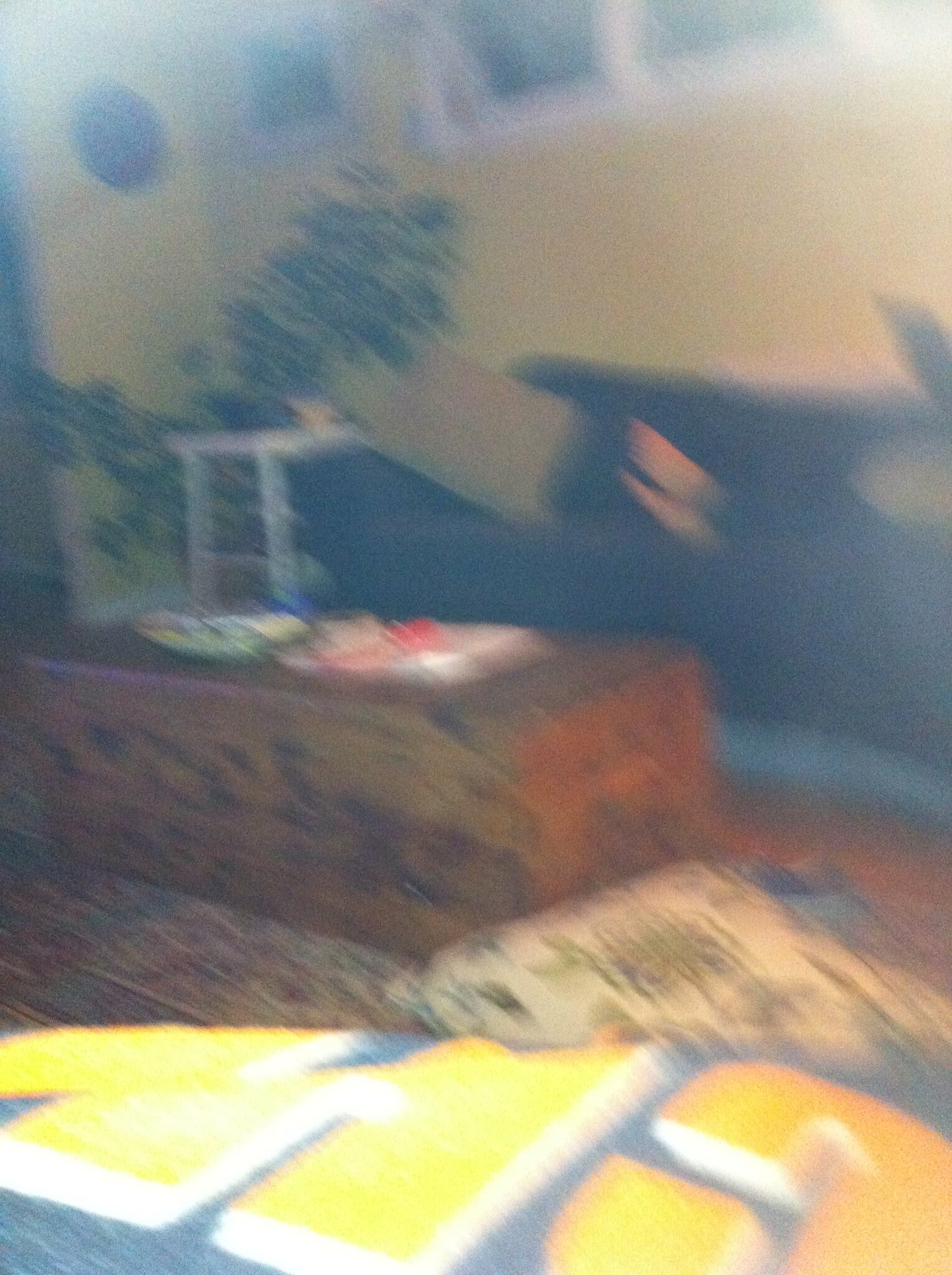This digital photograph, albeit extremely blurry and washed out, portrays a cozy interior scene of a living room, perhaps in a house. Dominating the middle of the room is a large, rectangular wooden chest serving as a coffee table, adorned with a few indistinct items, including a shallow decorative bowl and a stack of papers. Resting on a plush, oriental rug with a fancy golden design against a red backdrop, this chest is juxtaposed with a circular carpet that features yellow, 3D-like letters "C" and possibly "N" or "H" against a blue background. 

Against the yellow-painted upper wall, highlighted by a strip of darker blue below and trimmed with a white baseboard, stands a dark blue couch. The couch is accented with various colored pillows, some of which have spilled onto the floor. Above the couch, there are three transom windows, with at least one open, framed in white. The walls are adorned with a mix of paintings or prints, adding an artistic touch to the space.

To the left of the couch, perched on a white end table, is a four-foot-tall, healthy, and lush potted plant. Close by, a patterned pillow lies next to the chest. The blurred foreground suggests that this may be a photograph taken carelessly, possibly featuring the shoulder of the person who took it, clad in a gray shirt with letters "C" and "N" vaguely visible.